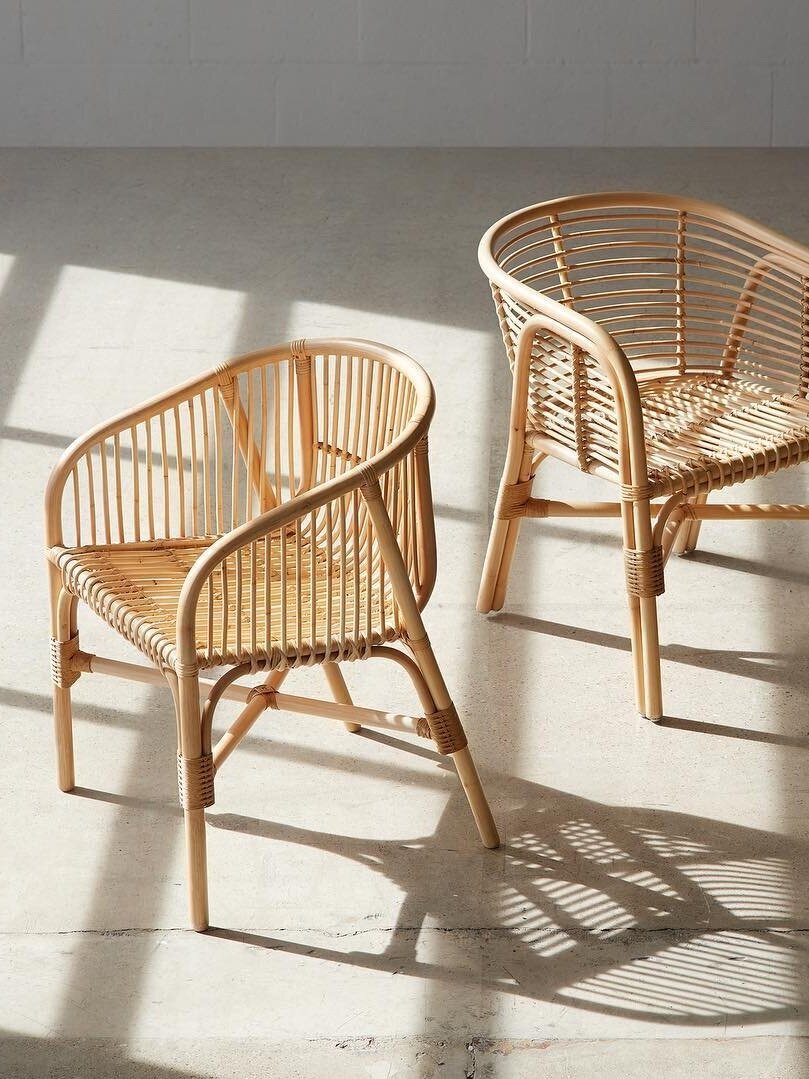The image depicts a minimalist indoor scene featuring two small, light brown wicker chairs without cushions. The chairs are positioned on a white, possibly concrete, floor against a backdrop of white-painted cinder brick walls. The front chair, facing left, sits in a sunny patch created by the sunlight streaming through a window on the left side of the frame. Behind it, the second chair faces more to the right, its right leg partially cut off from view. The chairs cast distinct shadows on the floor, with the sunlight illuminating vertical panels on the window, reinforcing the sense of a bright, serene atmosphere.